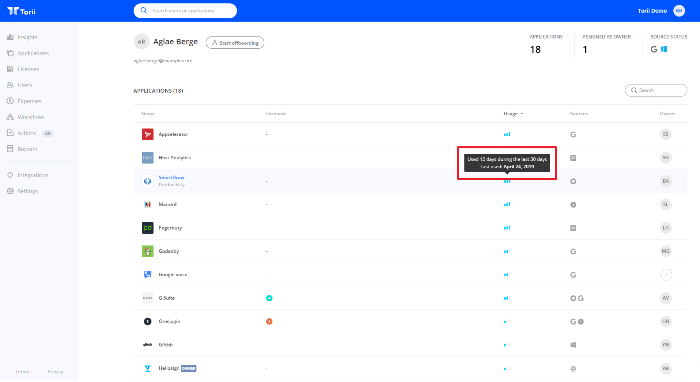On a white background, there's a blue rectangle at the center with the text "Tori and white" displayed prominently. Below, there's a search bar labeled "Agley" with the suggestion "Birch for Agley." To the right of the search bar, there's a gray circle containing the initials "AB" in black. 

Directly below this, the screen shows a section titled "Applications" with a figure of "18" next to it. Following this title, there's an organized list that resembles a chart. The list is divided into columns, one of which is labeled "Application" or "Applicator," while another column seems to highlight "New Replies" in blue text. However, the exact words were unclear. 

In the middle of the list, there's a cell with a blue word that is highlighted, though its content is not fully legible. Adjacent to this, a red rectangle encloses a smaller black rectangle detailing text about usage and timestamps. Specifically, there's a mention of "12 days used" and "20 days," with more text leading to the date "April 20th, 2024," although it also confusingly references "2004." 

On the left side of the screen, there is a vertical blue rectangle listing navigational options labeled as "Insights," "Applications," "Themes," and "Users."